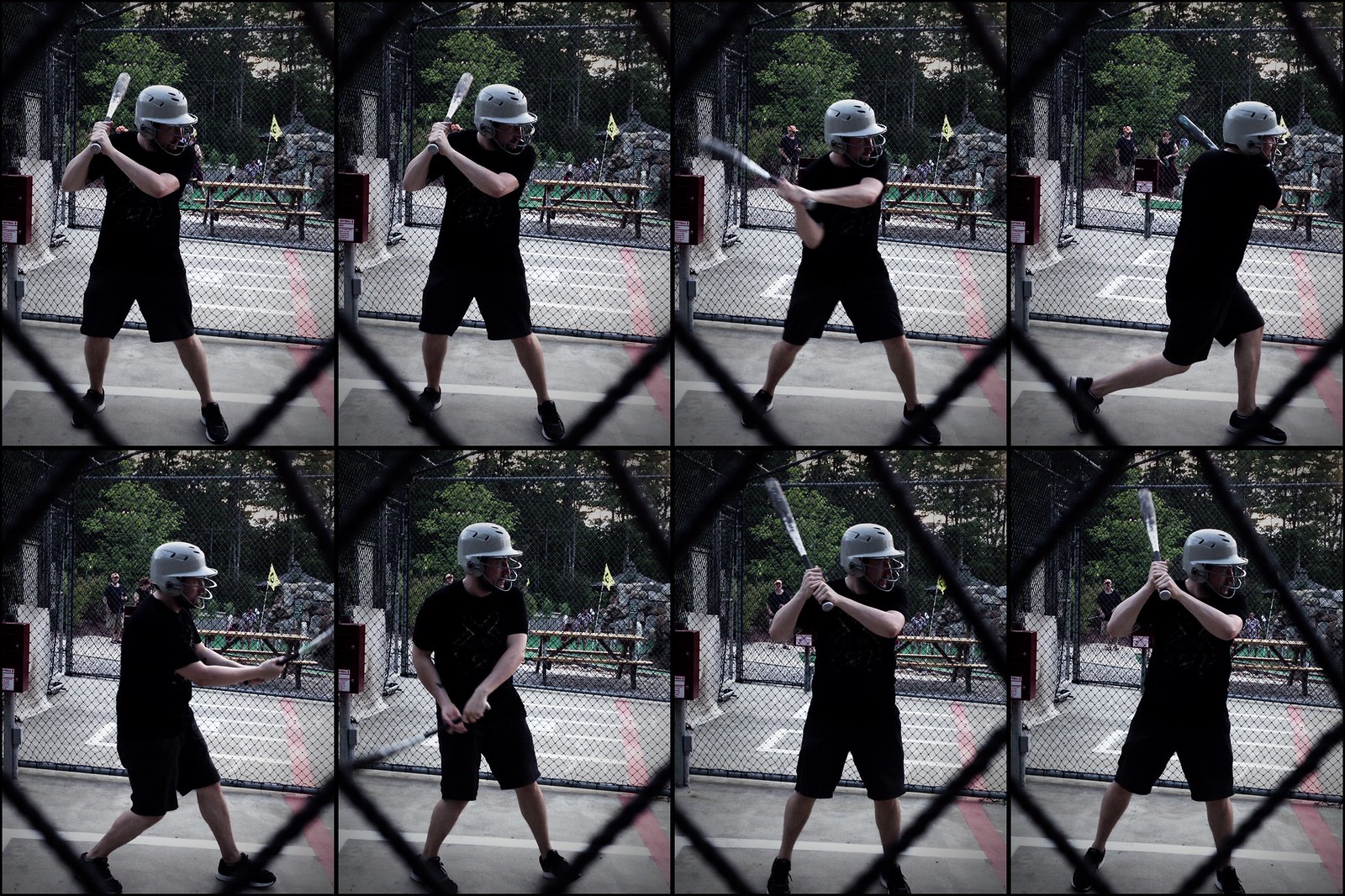This image is a detailed series of eight high-speed photographs, arranged in two rows of four, capturing the sequential motions of a baseball player swinging a bat in a batting cage. The scene starts with the batter in a ready stance, progresses through the swing, and concludes with the follow-through and return to the batting position. The player is outfitted in a gray helmet with a face guard, a black t-shirt, black shorts, and black shoes with white rims. He wields a silver aluminum bat showing signs of wear. Taken through a chain-link fence, these outdoor photographs also reveal a concrete base beneath the batter. Another chain-link fence is visible in the background, adding depth to this dynamic portrayal of athletic movement.